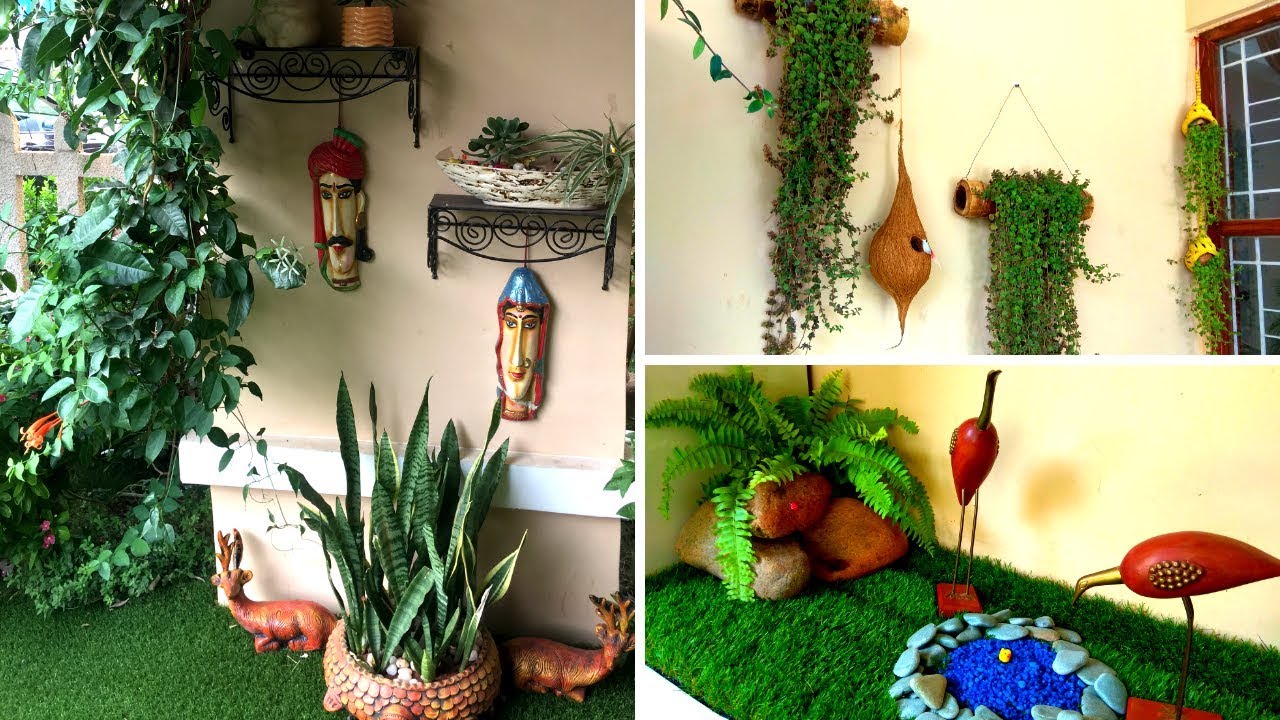This triptych showcases an indoor-like setting, possibly a deck or porch, adorned with a plethora of houseplants and artistic sculptures. The far-right photograph prominently features a collection of houseplants, including ferns and ivy, housed in various planters and black metal rod shelves. Sculptures resembling caricatures of people dangle from the wall, accompanied by a sizable planter on the green, astroturf-like floor, which also supports two clay deer sculptures. In the upper right, a bird's nest-like coconut structure hangs by strings, juxtaposed with two small yellow pots by a window, adding to the verdant ambiance. The central image reveals a beige wall backdrop with black metal shelving, showcasing painted masks—one of a man in a red turban and another of a woman in a blue shawl—with an ivy plant cascading over artificial green grass below. The composite imagery weaves a vivid tapestry of greenery, art, and whimsical sculptures, creating a uniquely inviting space.